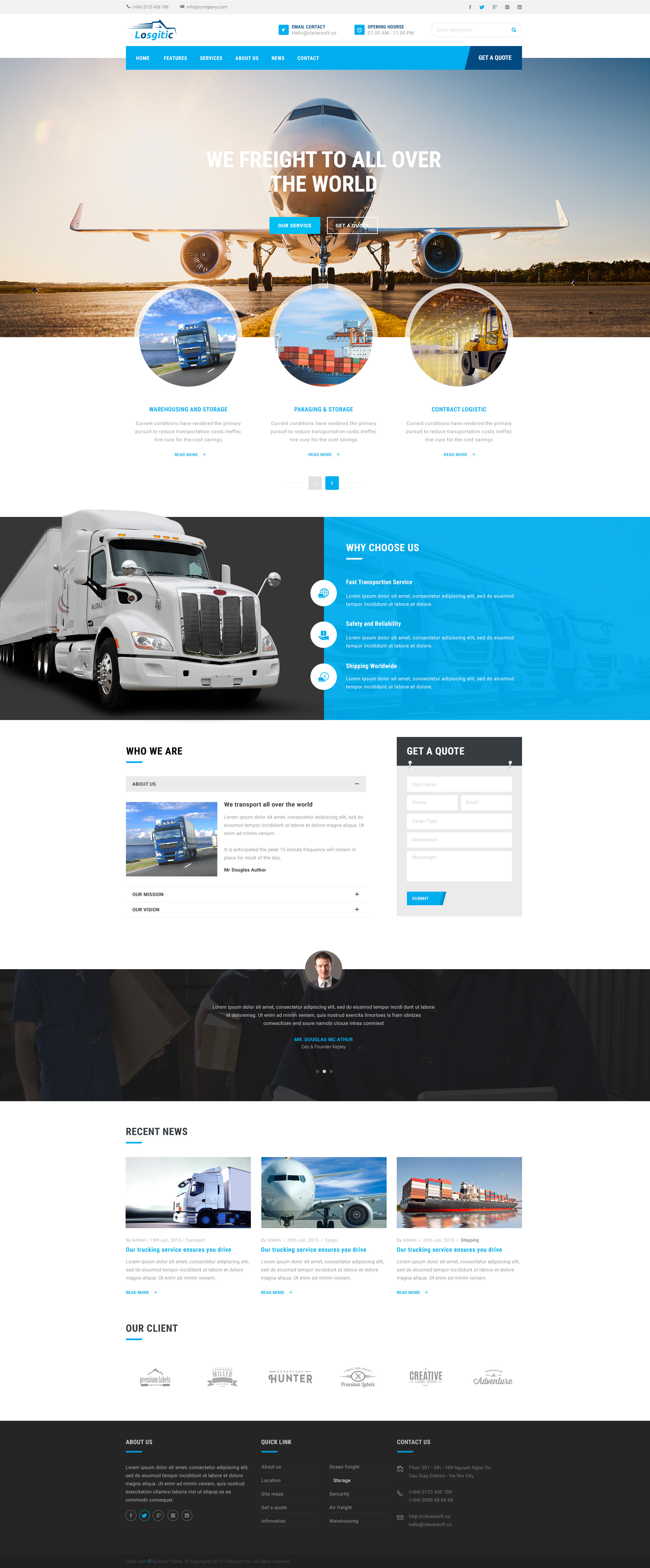The image is meticulously divided into four prominent sections. In the upper left corner, a logo is prominently displayed. Adjacent to the logo are two selectable options, all housed within a gray navigation bar, which also reveals there are five pages in total.  

The primary image captures a majestic upward view of an airplane, showcasing its engines and wings against a bright, cloudless sky. The horizon line sits low in the composition, emphasizing the expansive sky. Superimposed on this scene are three smaller, circular images: a blue Mack truck, some orange traffic pylons, and a yellow-and-black forklift truck. Overlaying the main image is the text, "We freight all over the world," flanked by two buttons – one solid blue, the other clear with a white outline. Beneath this, three paragraphs of text provide additional information, followed by a gray button and a blue button.

The following segment to the right of the airplane showcases an 18-wheeler truck on the left and a solid blue box on the right. Central to this section are three buttons, and white text is positioned strategically on the right-hand side.